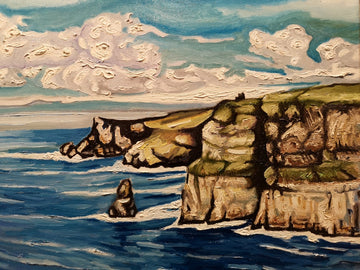This painting vividly captures a rugged coastline featuring a prominent landmass with steep cliffs that dramatically plunge into the ocean. The cliffs, composed of brown and white rocks, are topped with patches of green grass. On the left side of the headland, there's a gentler slope that seems climbable, contrasting sharply with the adjacent sheer cliff that ends in an upturned edge. In the ocean below, windblown waves crash powerfully against the rock formations that jut out from the water. The sky above is filled with thick, bumpy clouds, painted with a textured technique that gives them a three-dimensional presence. The backdrop sky is a blend of greenish-blue hues, enhancing the overall mood of this striking seascape.